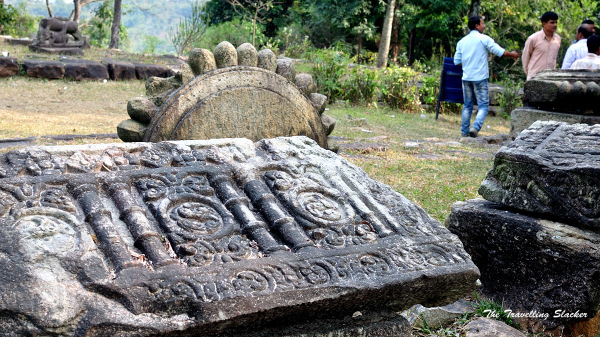The image depicts a scene set in what appears to be a rural, ancient site, possibly a temple or a circle of ruins. The focal point of the image is a large, dark, worn stone that resembles a gravestone or marker, featuring indecipherable engravings. This hefty stone is flanked by a circular stone with spines, adding to the mysterious and ancient atmosphere. In the middle ground, there are several other large, weathered stones, which might be remnants of a stone wall or part of the overall ruined structure. Lush green grass and bushes cover the foreground, with a backdrop of blue sky peeking through, suggesting a setting near a mountain forest.

On the right side of the image, a small group of three to four people can be seen standing on what might be a grassy pathway or a rough driveway, engaged in conversation. The group includes a man in blue jeans and a blue shirt, another man in a pink shirt, and a person in a white shirt. Their presence provides a sense of scale and modern contrast against the ancient stones.

Overall, the photograph evokes a sense of historical intrigue and cultural mystery, hinting at the remnants of an ancient civilization. The stonework, though fragmented and aged, suggests a significant past, potentially linked to Indonesian, Indian, or Polynesian heritage, inferred by the appearance of the individuals in the background.